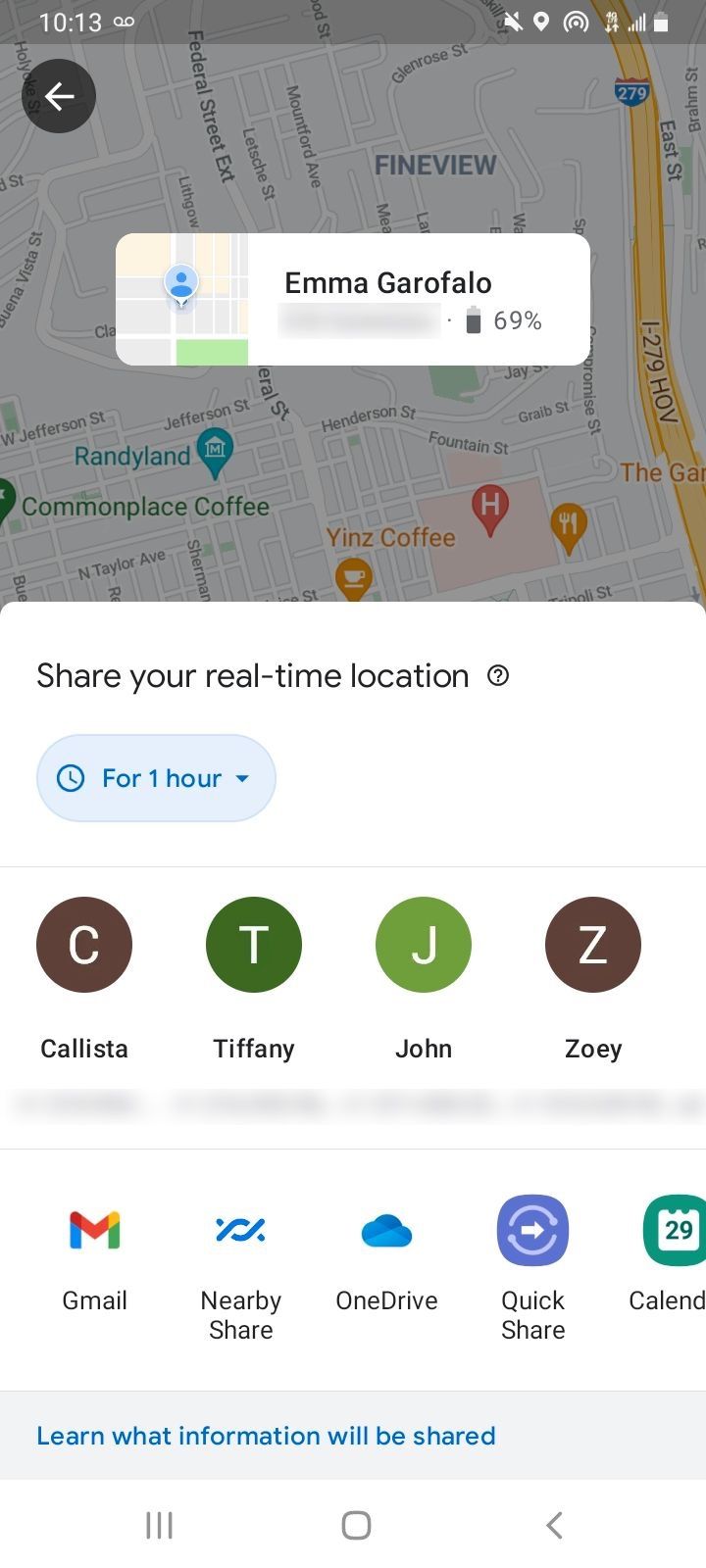A detailed screenshot of a map application is displayed, potentially from Bing Maps. At the top right corner, the battery icon shows about 80% charge, and next to it, the phone's signal strength appears at full bars. On the top left, the current time is 10:13. There is a circular icon featuring a left-pointing white arrow below the time.

Dominating the middle of the image is the map itself, prominently displaying the name Emma Garofalo. Adjacent to this name, in the bottom right section of the map, there is another battery icon showing a 69% charge.

The map features several labeled locations, including 'Randyland' and 'Commonplace Coffee' in the bottom left area, and 'Fine View' and 'Federal Street Exit' in the top middle region. 

Beneath the map, instructions to "share your real-time location" are shown. This is followed by an oval option labeled "for one hour" and a list of names: Calista, Tiffany, John, and Zoe. Further below, there are sharing options displayed as icons for Gmail, Nearby Share, OneDrive, Bookshare, and Calendar.